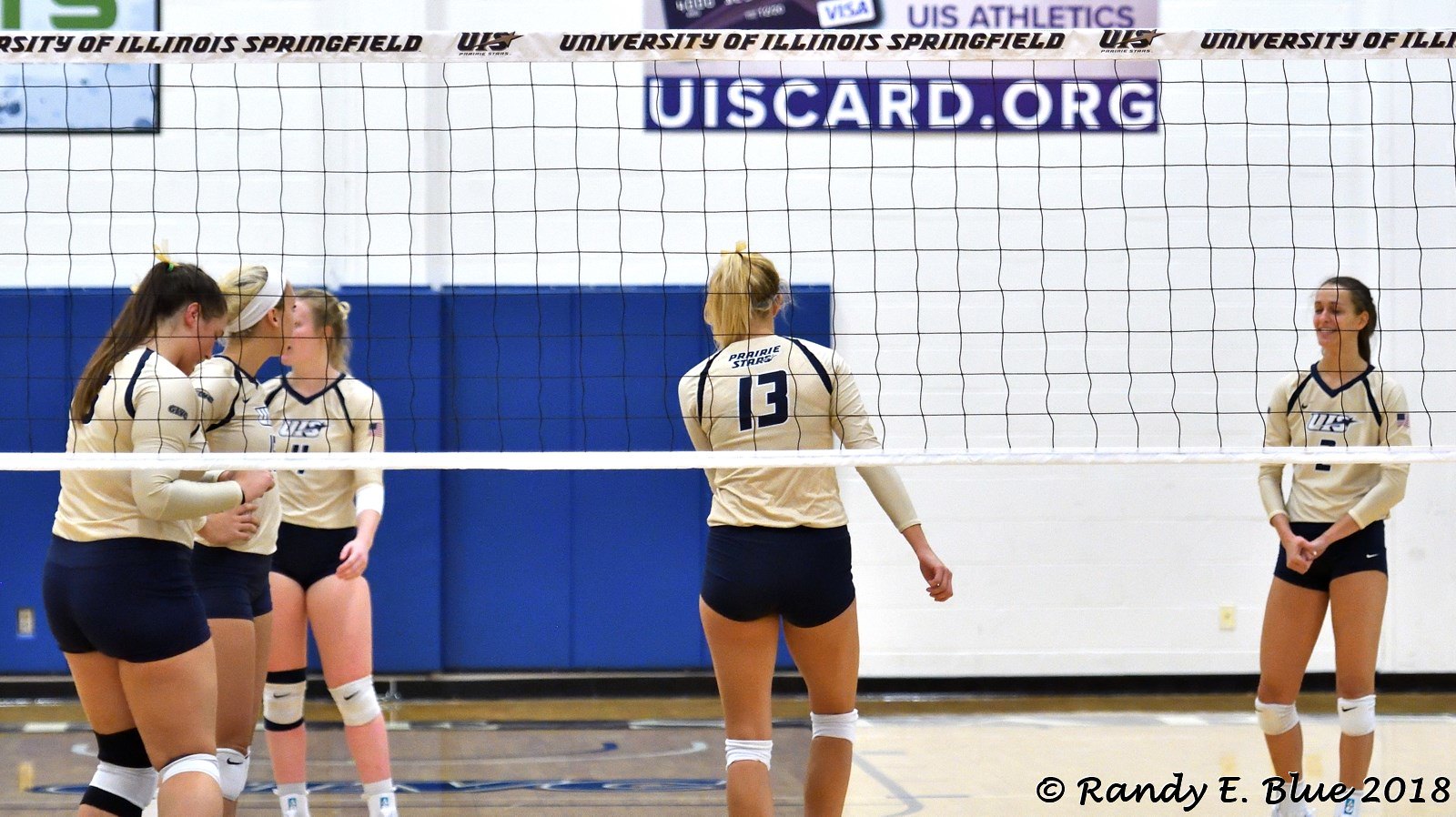In this detailed image, five young women are positioned behind a volleyball net inside a gymnasium, all dressed in white long-sleeved volleyball uniform shirts paired with dark blue shorts and white knee protectors featuring a logo. The team members' hair is neatly tied back in ponytails, with some notable differences: the woman on the far right, a brunette, has her hair pulled back, while to her left stands a blonde with the number 13 on her jersey, her back facing the camera. Next to her is another blonde with a ponytail, followed by yet another blonde wearing a ponytail and a white headband. To the leftmost position is a brunette with long dark hair, looking downward.

The gymnasium background reveals a white wall with various banners. A prominent one reads "UIS Athletics" with the logo of Visa and "uiscard.org." Another smaller banner in the top right corner is indiscernible. A blue padded section is visible on the left-hand side of the wall. Additionally, a strip bears the logo and the name "University of Illinois Springfield." The image's lower right-hand corner features a watermark or copyright marking from Randy E. Blue dated 2018. Overall, the scene captures a moment of focus and anticipation with the team poised to play on a brightly lit volleyball court.